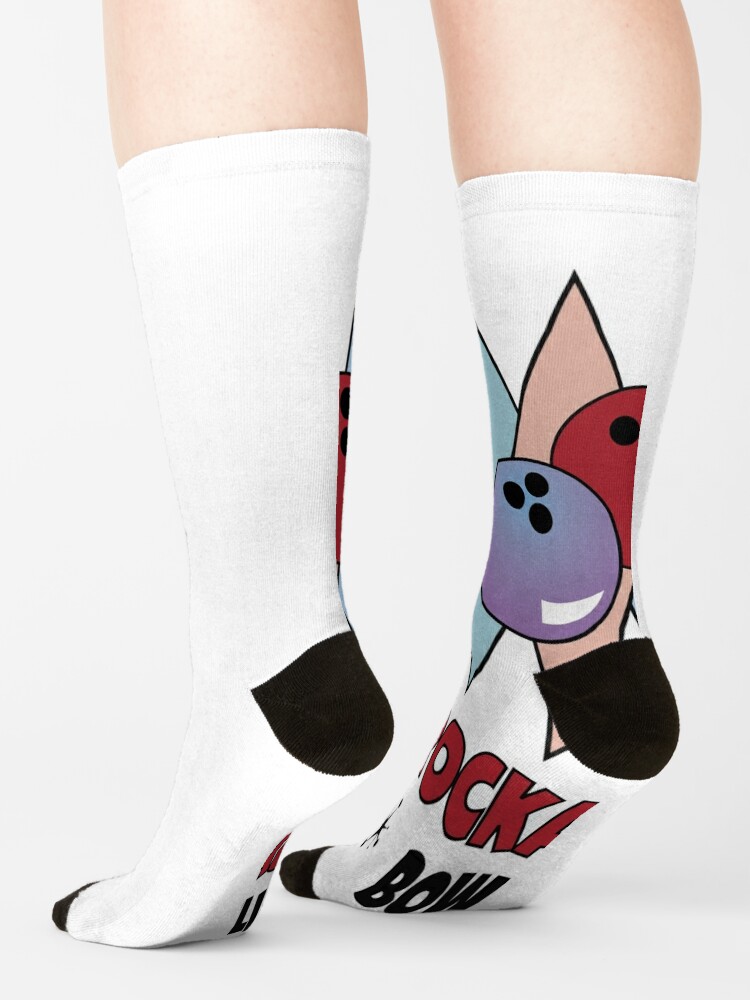The photo features a pair of high white socks with black toes and heels, seen on a person standing on tiptoe against a clean, white studio background. The image is cropped just below the knees, focusing on the legs and feet. There are illustrations on the inner sides of the socks: a purple bowling ball and a red bowling ball, along with partial red and black text that includes the letters "B-O-W" in black and "O-C-K-A" in red. The left sock's design is partially hidden, making it more visible on the right sock, contributing to a minimalistic and sporty aesthetic.